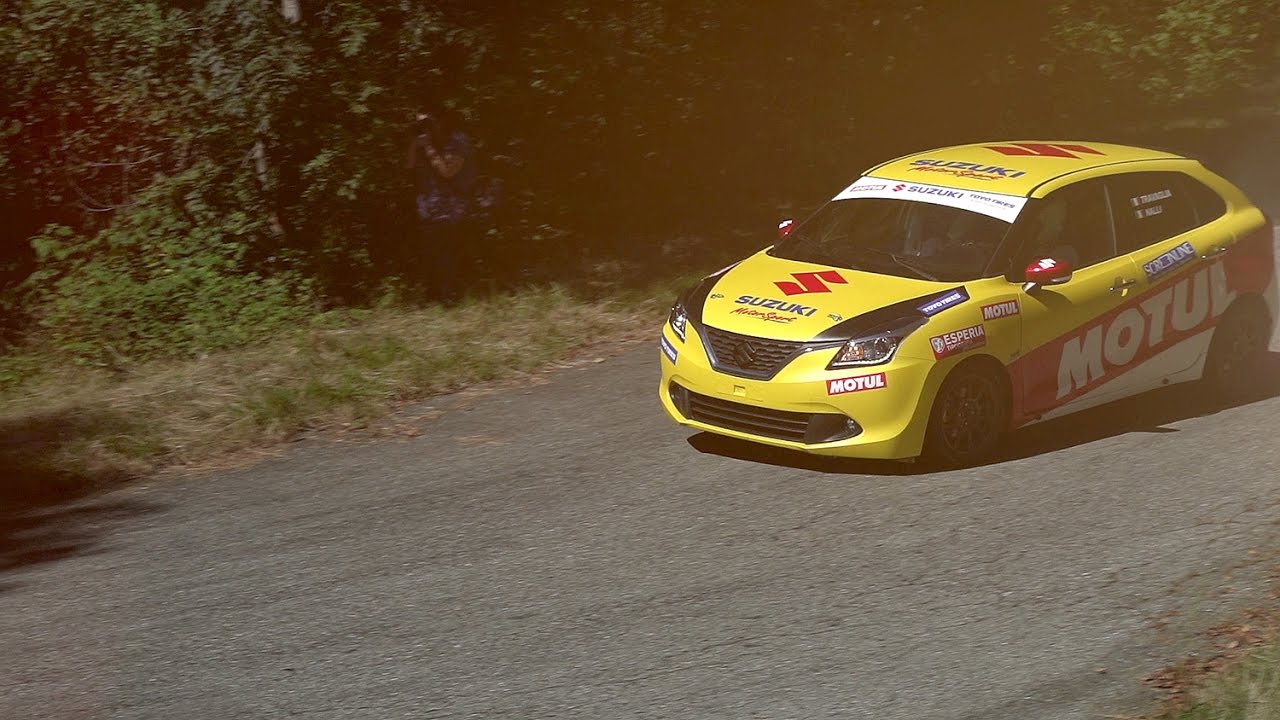In this daytime outdoor photograph, a bright yellow four-door race car, adorned with various sponsor logos and stickers, is parked alone on a desolate country roadway devoid of any markings. Prominently displayed on the hood in blue capital letters is "Suzuki," accompanied by a large red "S" both on the hood and the roof, enhancing its racing aesthetics. The side of the vehicle features a bold red stripe with the white capital letters "M-O-T-U-L," indicating a potential sponsor. The car's black grille, chrome door handle, and darkly tinted windows give it a sleek, polished appearance. Despite the deserted and worn road, the car stands out in vibrant contrast against the surrounding green grass and trees. The letters and numbers on the car, some red with white backgrounds and others in cursive, add to its detailed and dynamic look fitting for a race car.